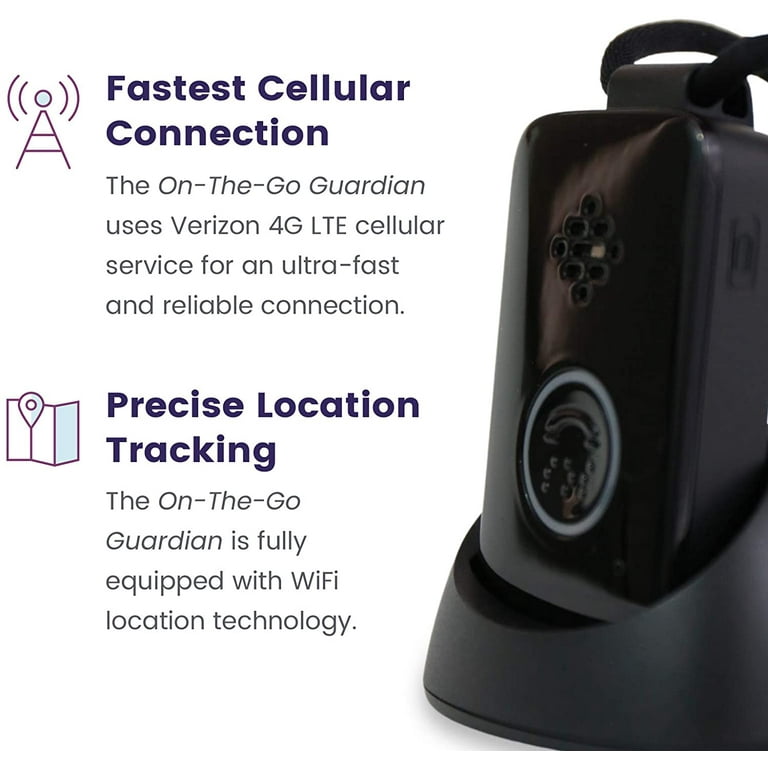The image appears to be a promotional slide with a white background, featuring a detailed advertisement for a product called the "On-the-Go Guardian." On the right side of the slide, there is a picture of a black rectangular device with a handle on top and various connection ports, possibly indicating it is a high-tech cellular device. The device is situated on what looks like a charger port. 

At the top left of the text section, prominently in bold dark black text, the tagline "Fastest Cellular Connection" is displayed with an icon resembling a cell tower surrounded by two curved lines on each side, illustrating signal waves. The text underneath, in unbolded font, states that the On-the-Go Guardian leverages Verizon 4G LTE cellular service to provide an ultra-fast and reliable connection.

Directly below this, another bold text reads "Precise Location Tracking" accompanied by an icon shaped like a teardrop with a dot in the center, reminiscent of a map pin. The supporting unbolded text explains that the On-the-Go Guardian is equipped with Wi-Fi location technology for highly accurate tracking.

Overall, the slide uses professional and clear formatting to highlight the main features of the product, emphasizing its swift connectivity and precise location capabilities.